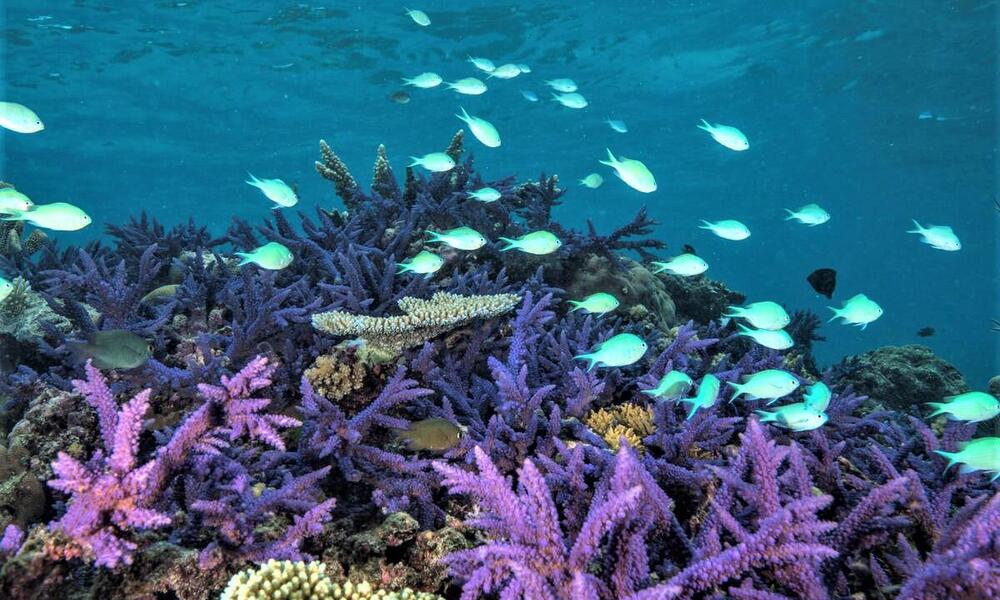This underwater photograph captures the vivid and bustling life within a coral reef. Dominating the scene are a school of neon-colored fish, primarily glowing green with subtle white accents, swimming uniformly towards the right. They are small, oval-shaped, and appear almost luminescent against the darker, somewhat murky blue water backdrop. The lower half of the image showcases a richly textured and colorful coral landscape. Predominantly purple, these corals branch out with clusters of round, globular formations, adding depth and complexity. Mixed within are patches of dark, almost black coral and other vibrant hues including yellow, brown, and beige. These diverse coral structures and the vibrant school of fish collectively create a striking and captivating underwater scene.